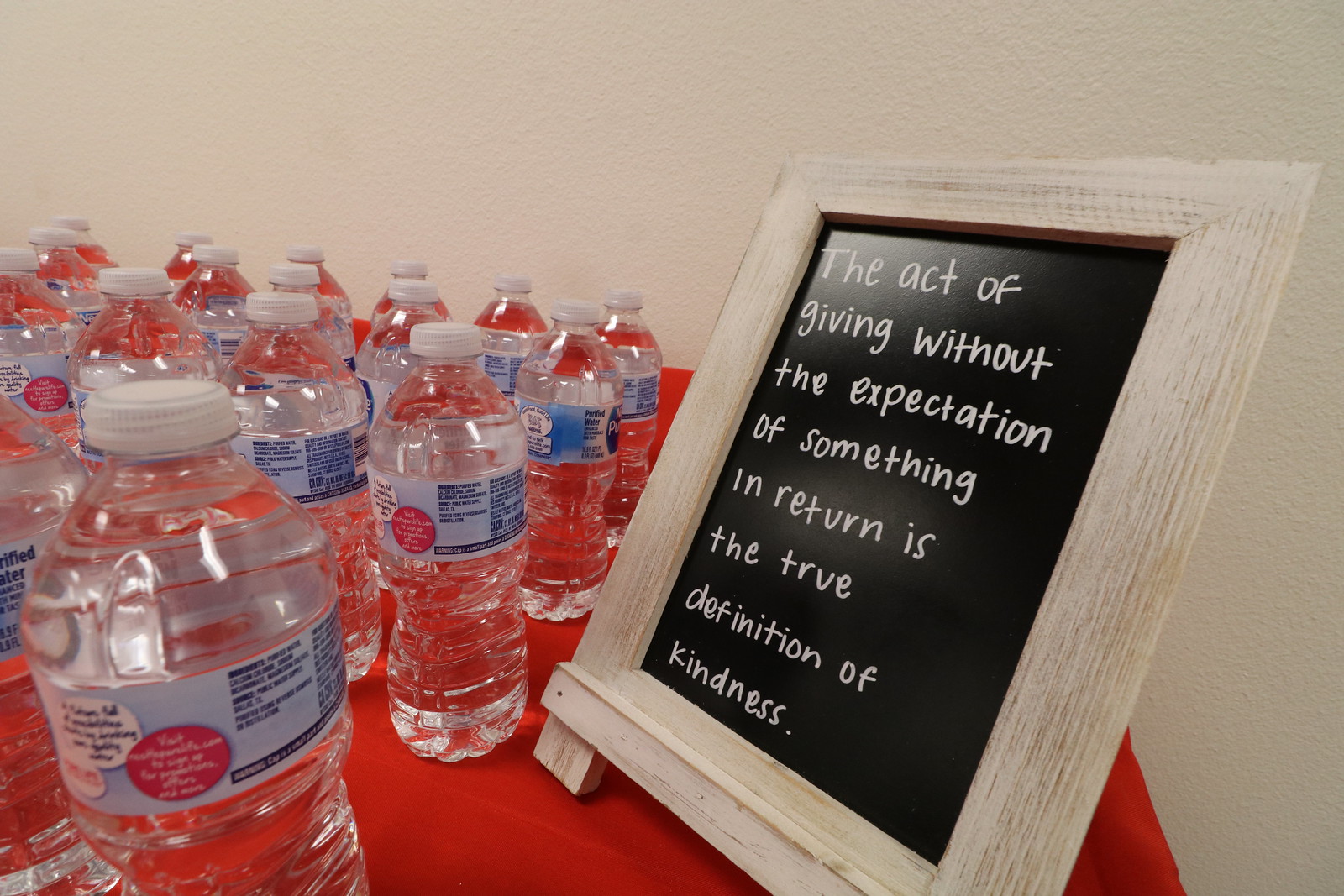The image is a detailed, photorealistic portrayal of a table draped with an orange-red fabric tablecloth, occupying the space from just right of center to the left edge of the frame. To the left side of the table, neatly organized into rows, are approximately 16 clear plastic water bottles, each adorned with blue labels featuring pink and white designs and dark blue writing. On the right side of the table stands a washed white wooden picture frame, angled slightly towards the left. The centerpiece of the frame displays a black background with white text that reads, "The act of giving without the expectation of something in return is the true definition of kindness." The wall behind the table is plain white, adding to the simplicity and focus of the scene, which evokes a sense of generosity and preparedness, possibly for an event or conference.